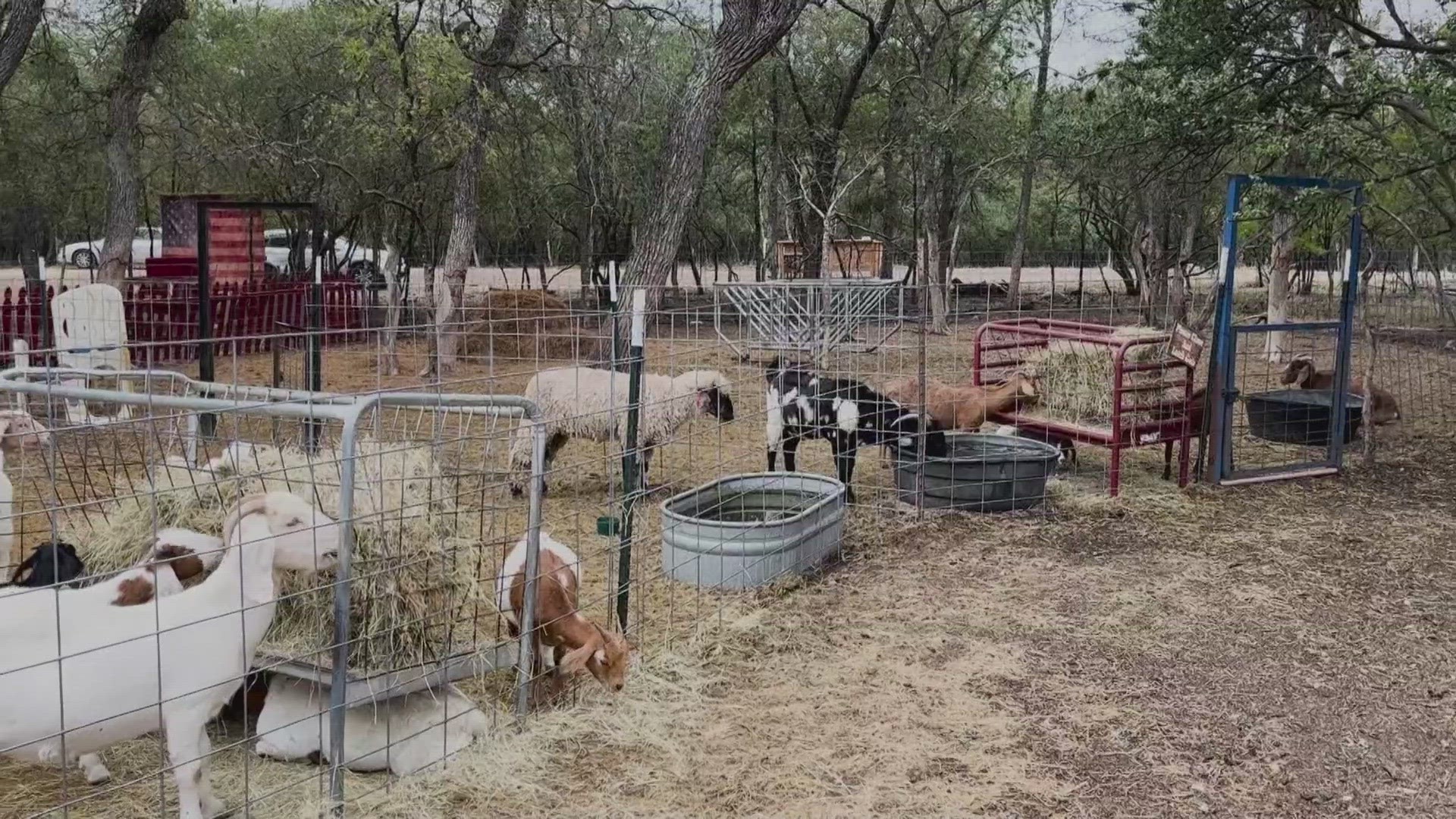The image depicts a rectangular, slightly wider-than-tall outdoor scene of what appears to be a petting zoo or a section of farmland showcasing livestock. Various fenced-in areas hold different types of farm animals, predominantly sheep and goats of various colors including white, brown and white, black and white, and completely brown. The enclosures are separated by small metal barriers, and some thicker metal structures likely represent gates. Inside the pens, large metal tubs of water can be seen, with a few animals drinking from them, and hay bales set in racks, with some animals nibbling on the hay. The ground is a mix of sparse, potentially dead grass and patches of bare dirt, especially towards the right side of the image. In the background, there are trees and more grassy areas, giving a slight impression of a park-like setting. Additionally, a few cars are visible in a parking lot at the back.